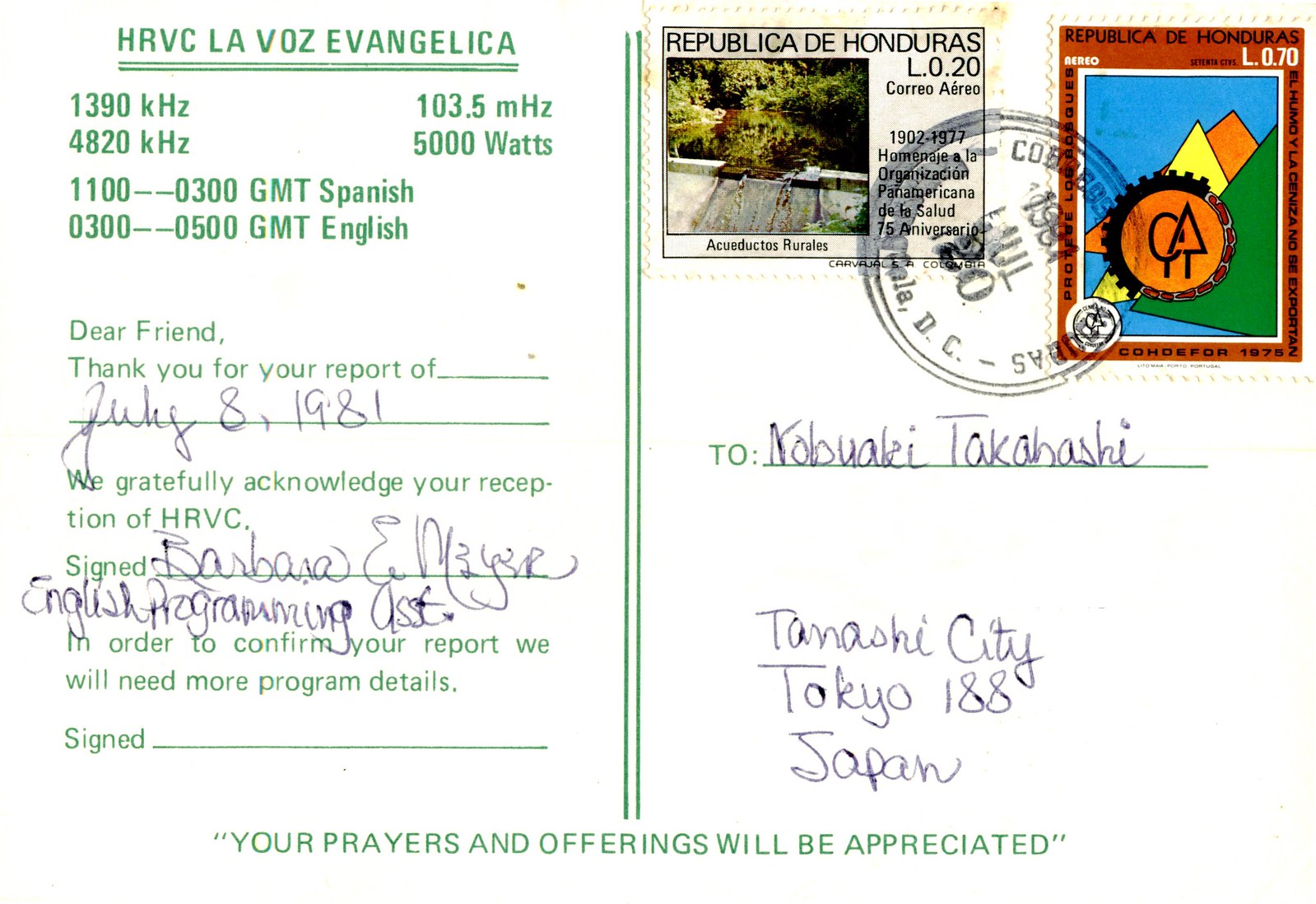The image depicts the back of a white postcard related to radio frequency, featuring vertical green lines dividing it down the middle. On the left side, at the top, it displays technical details including frequencies, wattage, and broadcast times in both Spanish (11 to 3 GMT) and English (3 to 5 GMT). Below, there's a handwritten message: "Dear Friend, thank you for your report of July 8, 1981. We gratefully acknowledge your reception of HRVC," signed by Barbara E. Mayer, English Programming Assistant. A note follows, requesting more program details to confirm the report. The bottom bears the inscription, "Your prayers and offerings will be appreciated" in green writing. On the right side, the postcard features multiple stamps from the Republic of Honduras; one depicts a wooded area with a deck, while another shows three multicolored triangles in a circle with an emblem. The postcard is addressed to Nobuaki Takahashi, Tamashii City, Tokyo 188, Japan, and is postmarked July 20, 1981.